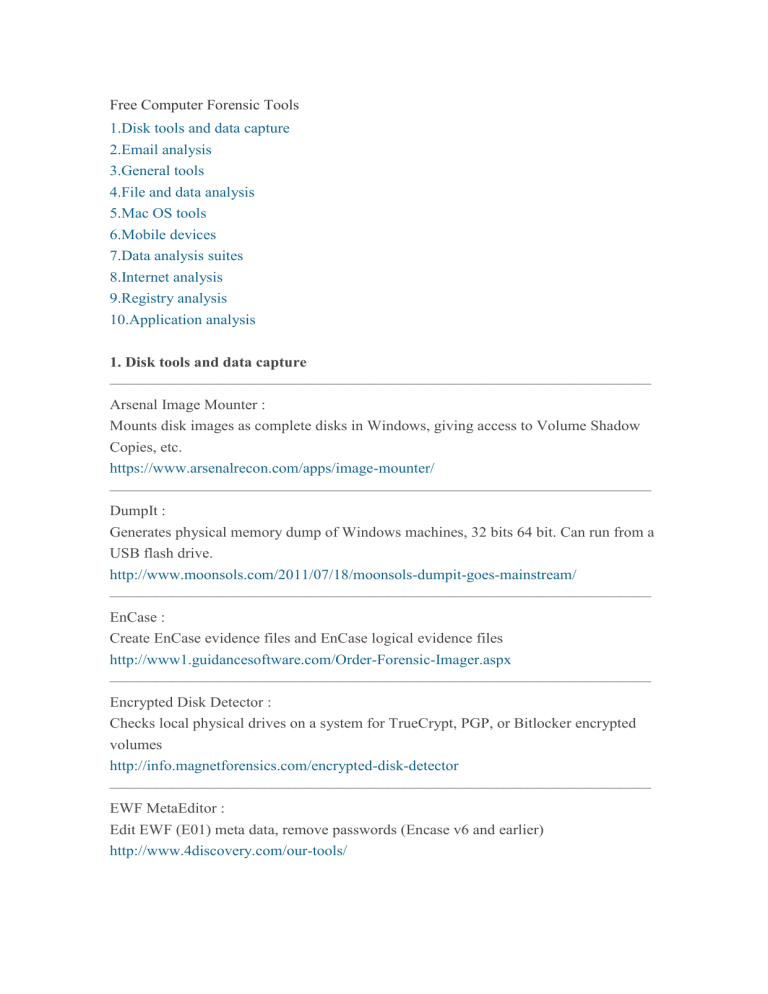**Image Description:**

At the top left corner of the image, the text "Free Computer Forensic Tools" is displayed in black Acera font. Below this heading, a numerically ordered list (1-10) in blue font (indicating clickable links) details various categories of forensic tools:

1. Disk Tools and Data Capture
2. Email Analysis
3. General Tools
4. File and Data Analysis
5. Mac OS Tools
6. Mobile Devices
7. Data Analysis Suites
8. Internet Analysis
9. Registry Analysis
10. Application Analysis

Following this list, another bold black Acera font heading reads "1. Disk Tools and Data Capture." Below this, a black line acts as a divider. 

In non-bold text, "Arsenal Image Mounter :" appears, followed by a description: "Mounts disk images as complete disks in Windows, giving access to volume shadow copies, etc."

Underneath this description, a blue clickable link is shown:
"https://www.arsenalrecon.com/apps/image-mounter/"

A long gray line at the bottom of the section serves as a divider.